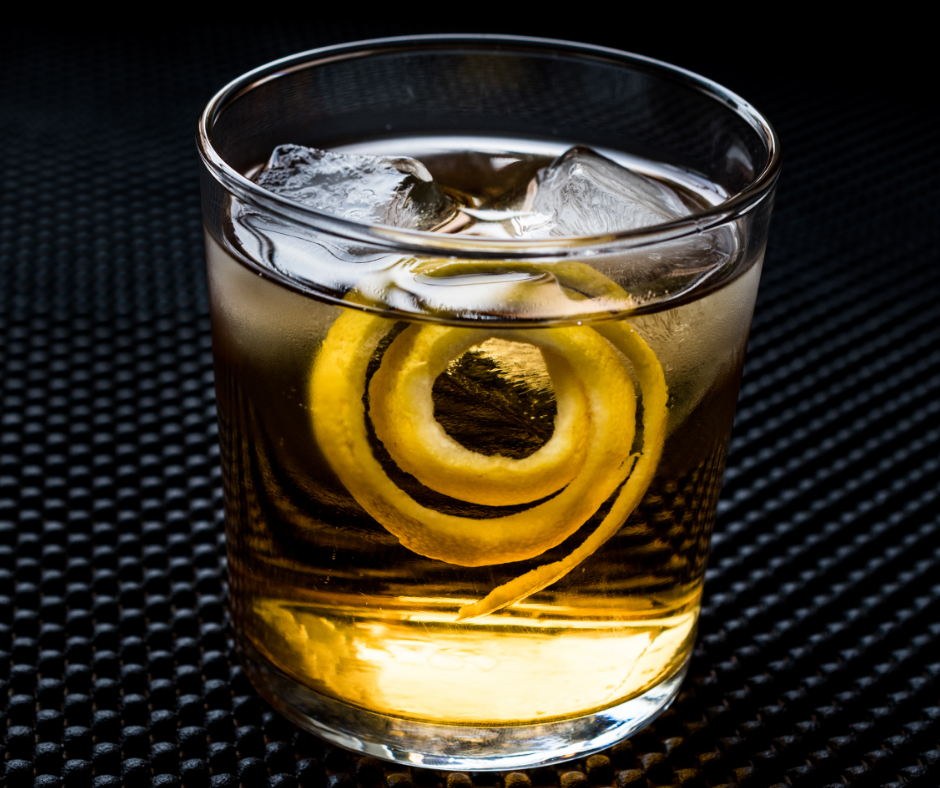The photograph features a clear, short tumbler-style glass commonly used for whiskey or bourbon, holding an amber-colored mixed alcoholic beverage. Within the glass, two perfectly cubed ice cubes float at the top, their corners softened slightly from melting. Adding a decorative touch, a lemon rind peel, meticulously cut into a spiral, rests in the front of the glass, enhancing the drink's visual appeal. The glass is placed on a black rubber mat adorned with tiny, bumpy structures resembling beads or bullet-shaped spongy shock absorbers, designed to prevent spills and provide grip. The background of the image is completely black, emphasizing the detailed presentation of the cocktail.